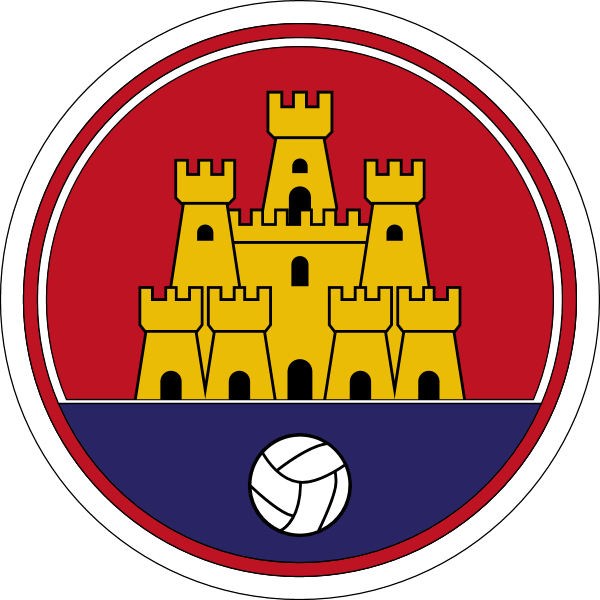This image showcases a circular emblem with a meticulously designed computer-generated graphic. The outer edge of the emblem features a sequence of thin lines: a black line, followed by white, and then a red line encircling the whole symbol. Dominating the top half of the emblem is a detailed yellow castle against a vibrant red background, complete with seven turrets, numerous windows, and six doorways, five at the base and one elevated above. The bottom half of the emblem contrasts with a deep blue background, centered by a white volleyball, symbolizing possibly a school or university sports team, distinctive for its animated and clearly defined design elements.